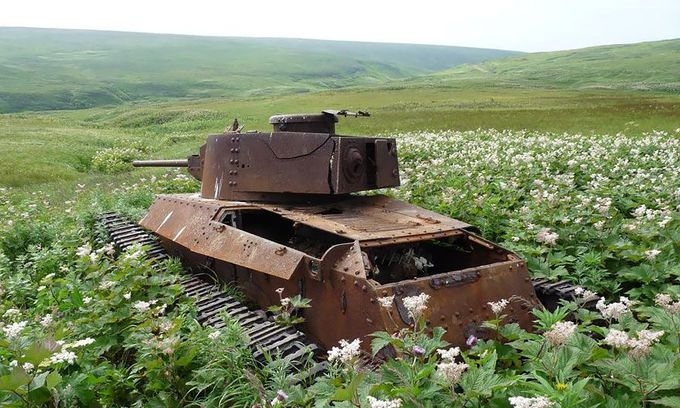In this photograph, at the center of the image stands a rusted, brown army tank with black tracks, surrounded by an expansive field of overgrown white flowers. The tank's cannon is pointed to the left, and there are noticeable open compartments and bolts on its left and middle sections, with treads visible at the bottom left. The scene is set outdoors during the daytime, framed by the lush greenery of the field and distant rolling hills that stretch into the horizon. The overall atmosphere is one of abandonment and nature's reclamation, as the tank appears hollowed out and engulfed by the thriving foliage, with no signs of human habitation in sight.